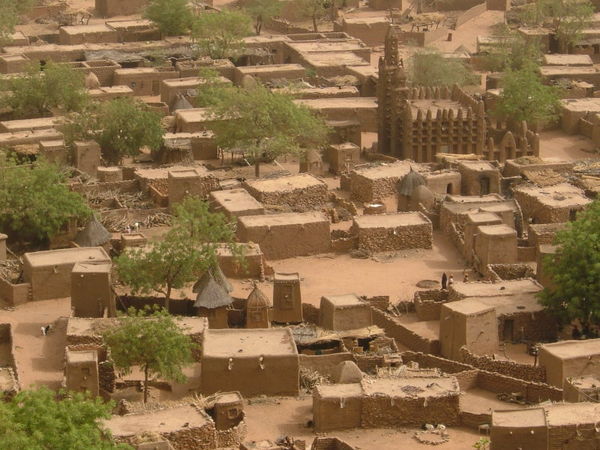The photograph captures a primitive-style mud village viewed from a higher vantage point, revealing an extensive arrangement of rectangular mud huts with courtyards and streets all in the same dried mud color. Some structures appear to be crumbling or in disrepair. The village is sparsely interspersed with green deciduous trees. Prominently in the upper right corner stands a unique church-like structure with three tall spires; the striking central spire flanked by slightly shorter ones. This edifice, built of pole-like mud columns joined in a gridwork pattern, is the tallest and most polished structure within the village. The overall scene is bright, and while figures are scarce, there are three small people visible in the middle portion of the photo, as well as a few animals scattered throughout.